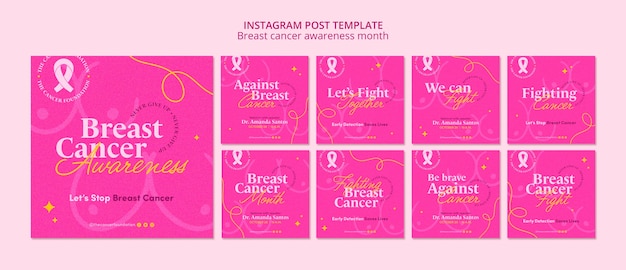The image is an Instagram post template designed to promote Breast Cancer Awareness Month. The template features a vibrant pink and purple color scheme. At the top of the template, in prominent brighter and darker pink text, it reads "Instagram Post Template." Below that, more text in a similar color combination announces "Breast Cancer Awareness Month."

The main section of the template is divided into a large square on the right and eight smaller squares adjacent to it. The large square, set in a dark pink background, includes two roughly drawn breast outlines—one located in the top right corner and the other in the bottom left. In the top right corner of this square, there is also a white ribbon symbol, representing breast cancer awareness. The text within this square reads "Breast Cancer Awareness" and includes a call to action: "Let's Stop Breast Cancer."

To the right, the eight smaller squares, each with the same pink and purple background, contain inspiring messages like "Let's Fight Together Against Breast Cancer." In each message, the last word is highlighted in yellow, while the preceding words are displayed in white text, effectively drawing attention and reinforcing the central theme of unity and action against breast cancer.